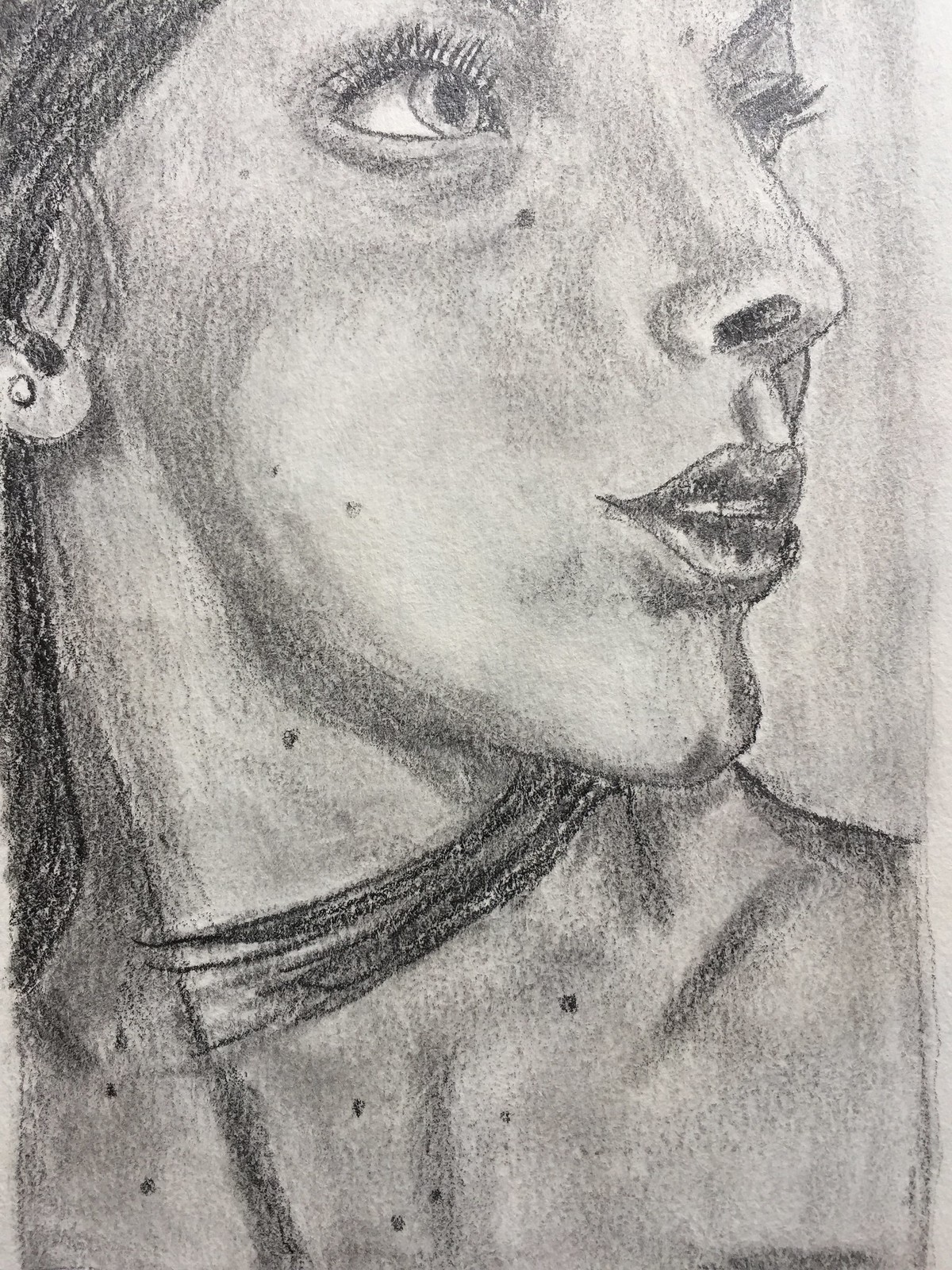This pencil-drawn portrait features a detailed side profile of a woman, showcasing an amateur yet heartfelt artistic effort. The woman has a pair of light-colored eyes, although they appear slightly too far apart, hinting at a novice artist’s attempt. Her long black hair elegantly cascades down her back with a few strands thoughtfully pulled over her neck to rest gently on her chest. She wears a simple stud earring, which accentuates her understated elegance. Her facial features are meticulously drawn—the nose is well-formed, and the mouth, though somewhat pointed at the corners, conveys expression. Her cheeks appear slightly rounded, adding a touch of softness to the depiction. A sprinkling of freckles adorns her neck, chest, and face, lending a touch of realism. The artist's use of a dark pencil brings depth and contrast to the drawing, highlighting the woman’s natural beauty and the artist’s attention to detail.